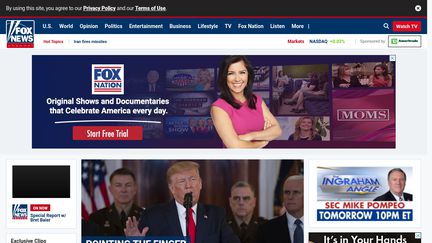This image, sourced from the Fox News website, features a prominent black bar spanning the top of the page, with white text situated in the top left corner. Directly beneath this black bar is a blue bar extending across the screen.

On the left side of the blue bar, the Fox News logo is prominently displayed. The logo is a square with a white outline, a blue background, and the words "Fox News" in white, accompanied by a red underline.

To the right of the logo on the blue bar, there is a series of white text links, which include categories like "US," "World," "Politics," "Entertainment," "Business," "TV," and an additional "More" section.

Centrally located on the page is a banner featuring a promotional message: "Original shows and documentaries that celebrate America every day. Start free trial."